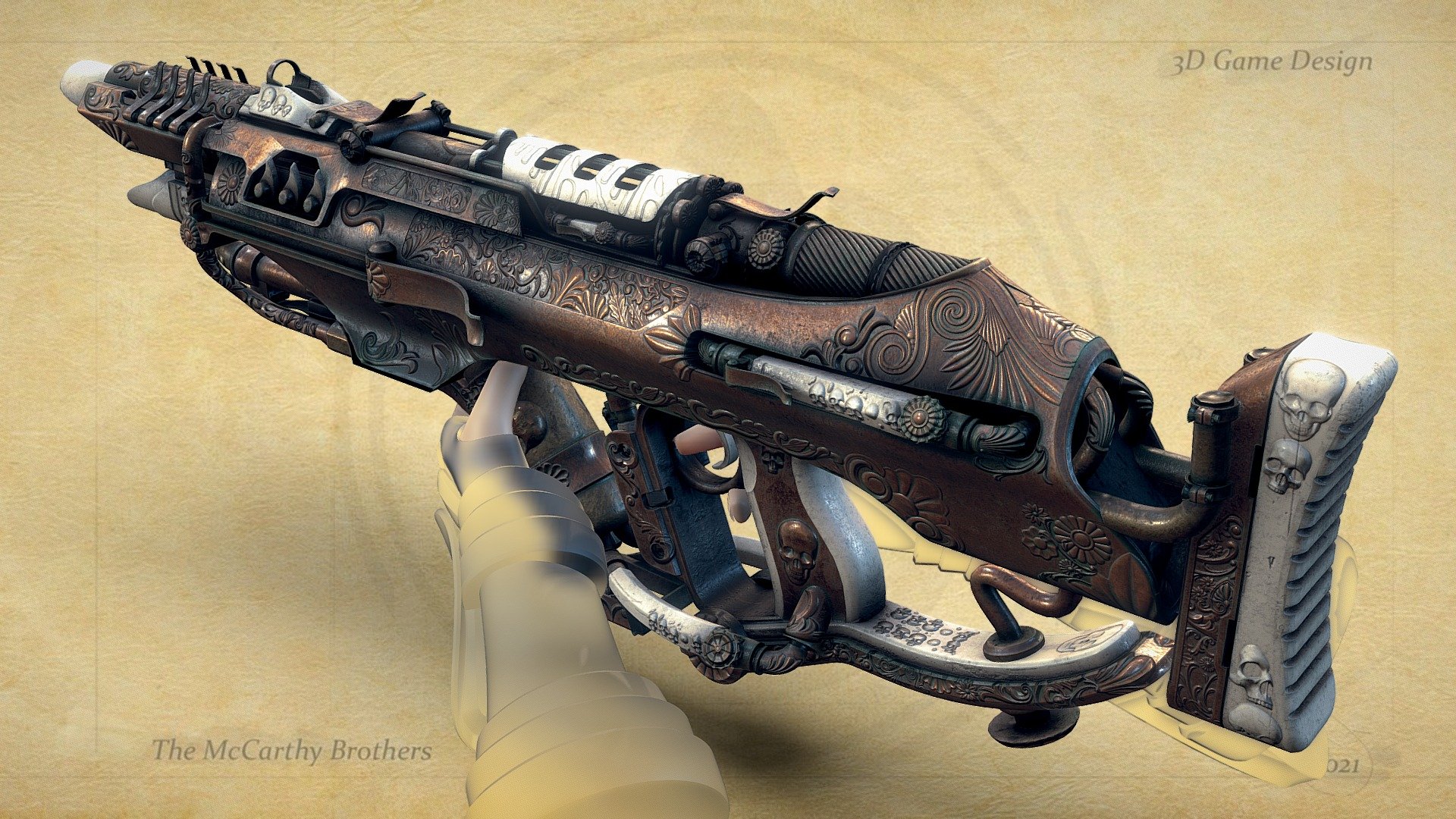This detailed image features a highly ornate, 3D-rendered, steampunk-style rifle, prominently displaying intricate designs and modifications. The caption "3D game design" appears in the top right corner, indicating its purpose within a video game environment, while "The McCarthy Brothers" label at the bottom left suggests the creators of this elaborate digital artwork. The gun itself is a complex blend of dark brown and black metals, adorned with silver and white trims. It boasts numerous flourishes, such as precise flower engravings and a highly detailed white shoulder brace embossed with skull designs. Additional steampunk elements include exposed wires, tubes, ornate carvings, heat vents near the muzzle, and multiple chambers and compartments not typically found on traditional firearms. A left hand, seemingly human, holds the gun, although the main focus remains on the weapon's elaborate design. A script notation "Page 321" is also visible at the bottom right, adding to the detailed and immersive presentation of this impressive 3D model.